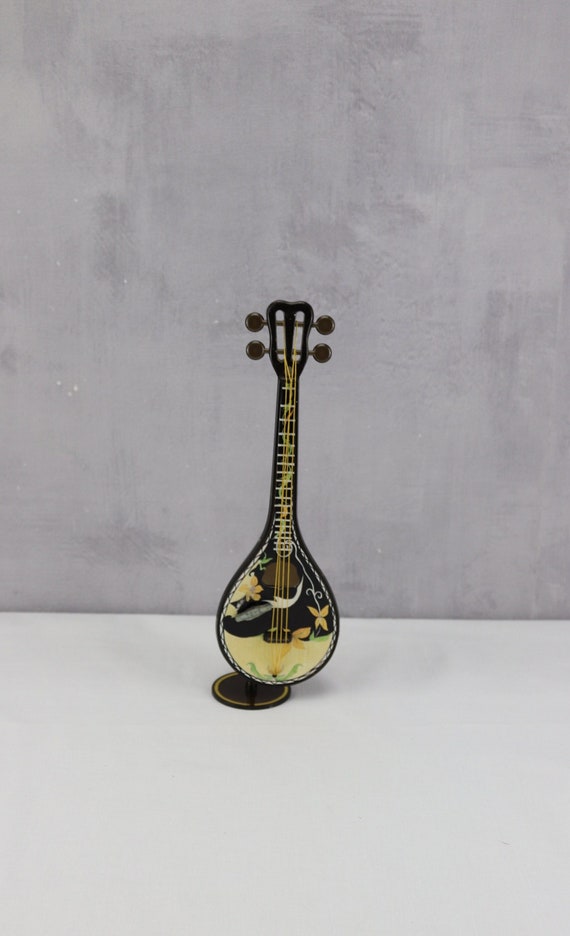The image depicts a black mandolin, or possibly a similarly sized stringed instrument, characterized by a rounded base and a narrow neck with four tuning keys. It is mounted upright on a black and yellow stand, set against a stark gray, possibly concrete, wall background. The mandolin features an intricate and colorful painted design, showcasing yellow and orange flowers with accompanying green vines, and potentially a white figure resembling a swan or butterfly behind the strings. The instrument itself appears to be smaller than a guitar and is displayed without anyone playing it, emphasizing its decorative and artful presentation.